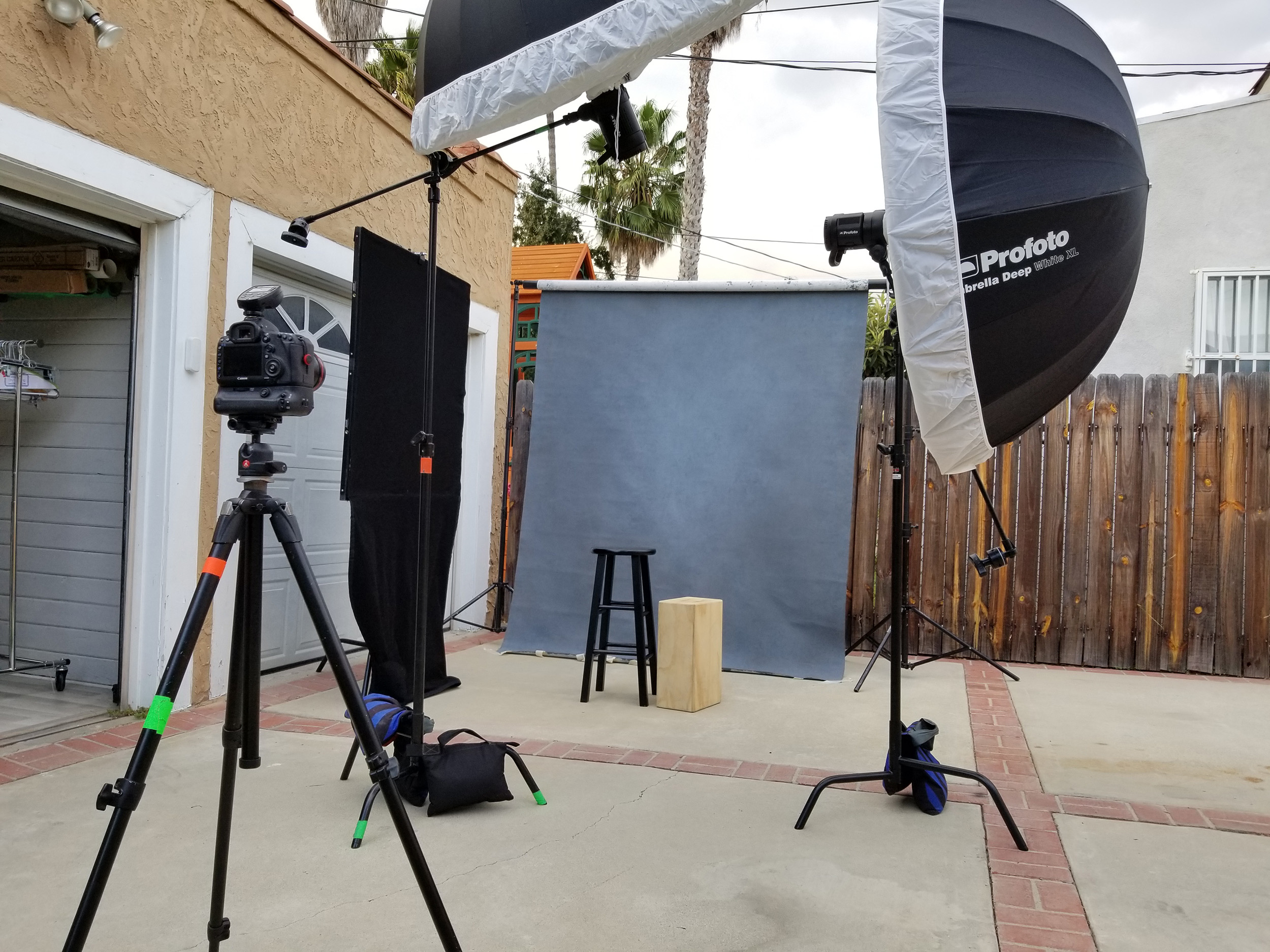This image depicts a well-prepared outdoor photo shoot set up in what appears to be a residential driveway, potentially located in California given the presence of a palm tree in the background. The scene is overcast with gray skies, adding a diffused lighting effect. The ground is concrete, divided by red brick separators. Central to the image is a digital video camera mounted on a tripod, positioned towards the left middle of the frame and pointing straight ahead. 

In addition to the camera, there are multiple pieces of professional lighting equipment. An umbrella labeled "Profoto Deep White XL" in white letters on its black exterior is notable. Another umbrella is partially visible at the top of the image, indicating additional light sources. 

The setup also includes a roll-down backdrop which is gray, placed behind a black stool and a large piece of wood approximately 8 by 8 inches in size. The lighting and camera equipment are meticulously arranged, suggesting meticulous preparation for the photo shoot. The setting, featuring a garage door on the left and surrounded by residential elements, underlines that the shoot is taking place at someone's home.